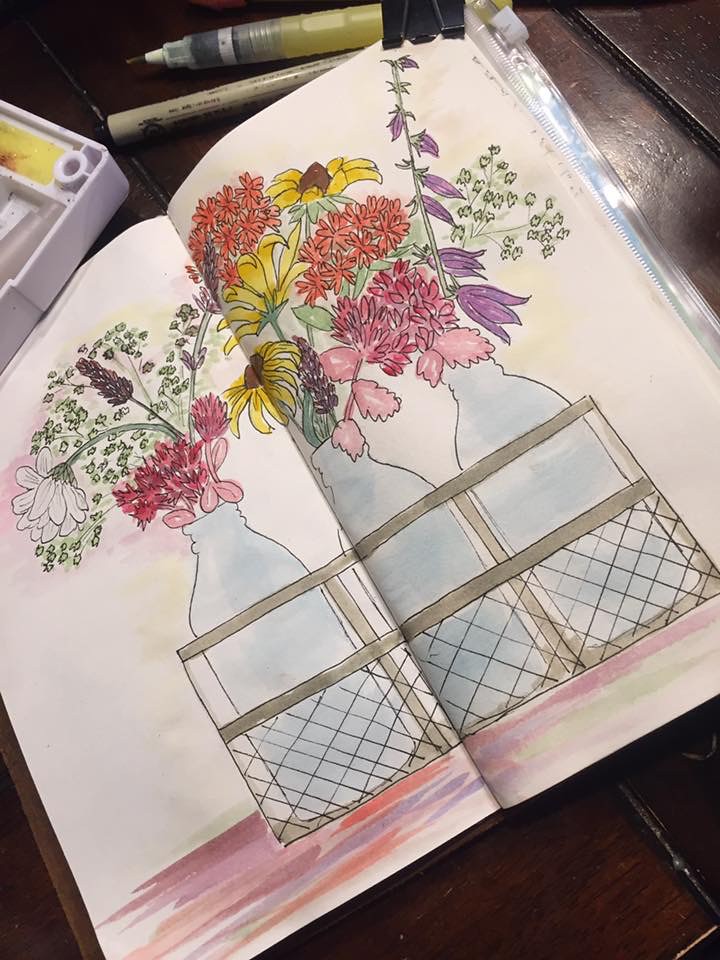On a small, brown-tiled tabletop framed with wood, sits an array of artistic materials and decorative elements. A plastic holder, designed to organize art supplies, contains various coloring pencils and pens. An open book, spread across the surface, showcases a beautifully detailed illustration, inviting creativity and imagination. Adjacent to the book is a gray wire basket holding three white, vintage-style milk bottles. Each bottle is filled with an assortment of vibrant flowers: delicate blue blooms, small yellow flowers, striking red and pink petals, large yellow flowers with brown centers, and a tall, elegant purplish flower, all harmoniously arranged to create a lively and colorful bouquet.